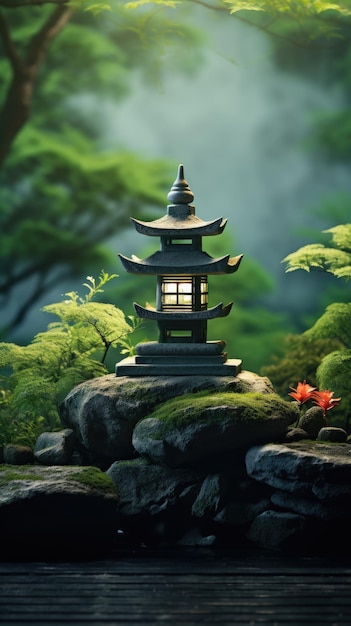This detailed AI-generated image portrays a serene, miniature Japanese garden scene. Central to the composition is a pagoda-style lamp, illuminated from within by a warm yellow light shining through its paper windows. The lamp, which has a square base and three progressively smaller, curling layers topped with a pointed cone, rests on a large, moss-covered stone amidst several other mossy rocks. Small green plants with jutting leaves and two red flowers add vibrant touches, balancing the dominant greens. This tranquil arrangement appears to be set in a shallow body of water, with layered stones extending out to the sides. The backdrop features an out-of-focus forest, enhancing the natural, peaceful ambiance of the scene.